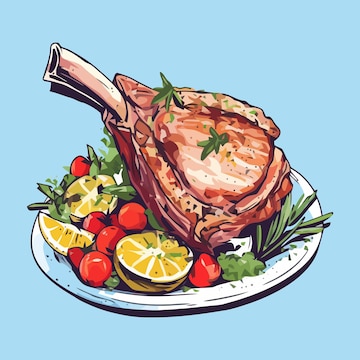This detailed painting, likely created with digital graphic tools or watercolors, depicts a succulent lamb chop entrée, meticulously presented on a white platter set against a light blue background. The lamb chop, cooked to a tantalizing brownish-red hue, features a prominent bone tinged with reddish and white tones. Adorned with vibrant green rosemary leaves and a mixed green salad, the dish is further embellished with juicy cherry tomatoes and zesty lemon slices. The artistic representation captures the dish's essence with rich details, highlighting the textures and colors of the ingredients used, creating an appetizing visual feast.